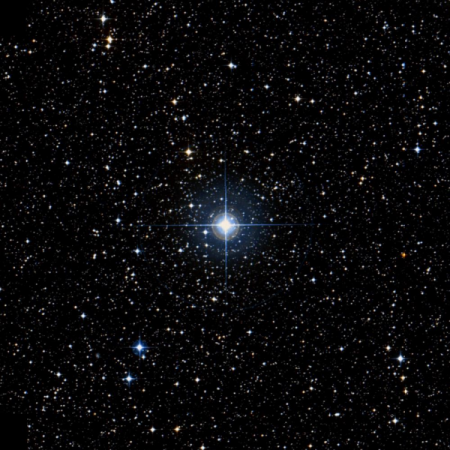This square image captures a detailed and mesmerizing view of the night sky, set against a deep black background. Dominating the center is a dazzling, diamond-shaped object that evokes the brilliance of a radiant star, adorned with a striking blue-tinted lens flare effect that forms an 'X' pattern. Surrounding this centerpiece, there is a glowing circle of light, emphasizing its intense brightness, which contrasts with the numerous smaller, twinkling white stars scattered across the entire frame. These smaller stars, some of which appear as dim diamonds and tiny white circles, create a celestial tapestry that enhances the impression of gazing into outer space. Notably, the lower left of the image features a few stars that are slightly brighter, yet still outshined by the central luminary, which exudes a captivating, almost ethereal glow.